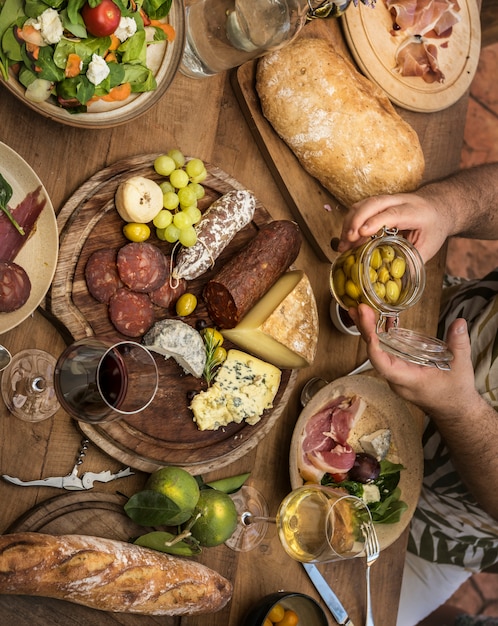This detailed overhead photograph captures an abundant charcuterie spread on a table, showcasing a diverse selection of food. Central to the image is a wooden platter brimming with a variety of items: a large wedge of cheese, blue cheese, a sprig of rosemary, two types of sausages (one sliced), grapes, a banana, and a few limes. Surrounding the platter are complementary dishes including two loaves of bread—a baguette and a wide peasant loaf—each on individual dark cutting boards. A bowl of fresh spinach salad, accented with carrots, a single tomato, and possibly artichoke hearts, is visible in the upper left corner. Two glasses of wine, one red and one white, are placed near the food.

A man, identified by his hairy forearms and possibly a black and white shirt, is seen holding an open jar of olives and has a plate containing a small salad and slices of ham. The table also features a corkscrew and a pitcher of water, enhancing the dining setup. The dark brown wooden table serves as a rustic backdrop for this visually appealing feast.